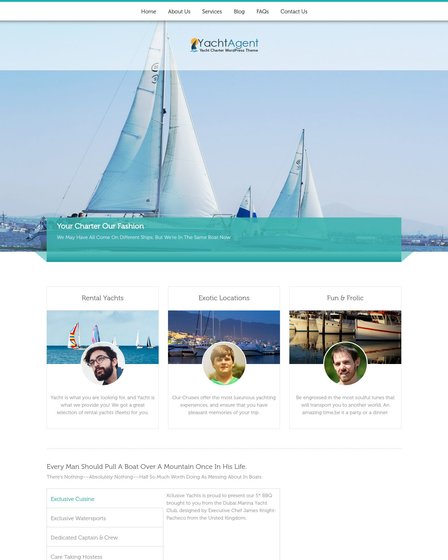The image is a screenshot from the Yacht Agent website. At the top of the website, there's a navigation menu set against a white bar with gray text, displaying the options: Home, About Us, Services, Blog, and Contact Us. The central image features three sailboats gracefully gliding through the water. One of the sailboats is prominently heading towards the left of the screen, offering a clear view of its side.

Overlaying this picturesque scene is the Yacht Agent logo and text, prominently displayed above the sailboats. Below the sailboat image, there's a translucent green banner with white text that reads, "Your Charter, Our Fashion." Further down, the website showcases three content boxes. Each box includes a title and an image of a person's profile picture. The titles of these boxes are Rental Yachts, Exotic Locations, and Fun, though the last word is somewhat obscured.